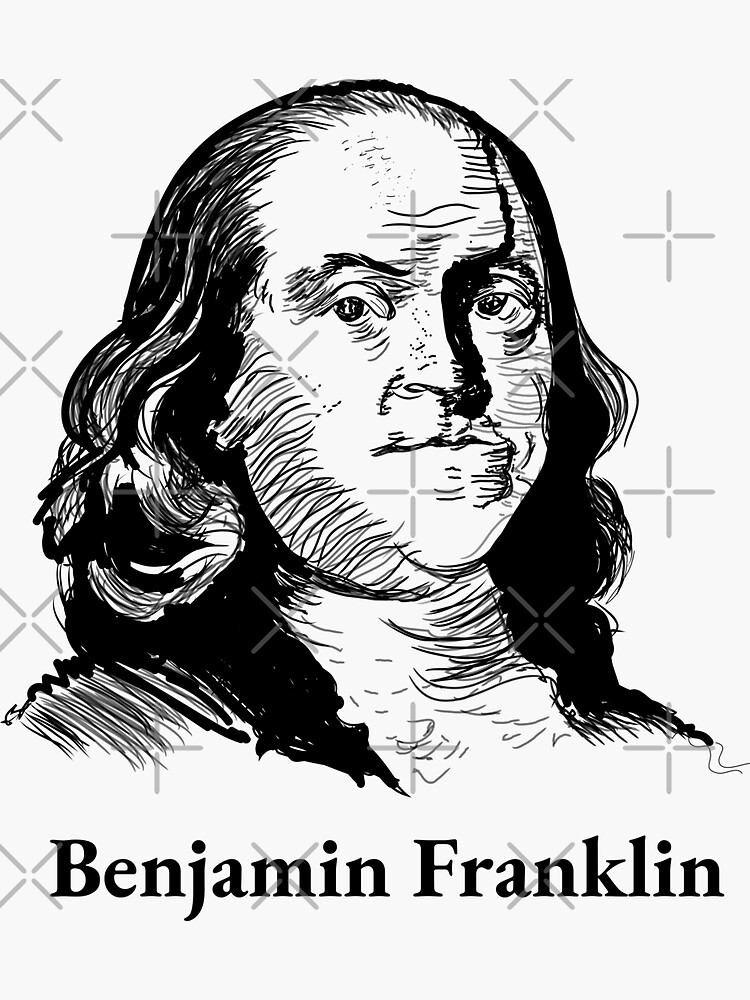This is a detailed black-and-white sketch of Benjamin Franklin, facing the viewer with a contemplative expression. His balding round head is accentuated by shoulder-length, wavy hair, with the right side mostly in shadow, adding depth to the portrait. The artwork features subtle gray cross patterns overlaying the image, creating a textured effect reminiscent of watermarks. The background is entirely white, emphasizing the stark, monochromatic nature of the drawing. Along the bottom left corner, in clear black font, the name "Benjamin Franklin" identifies this iconic historical figure. His robust yet composed demeanor is captured expertly, suggesting the intelligence and strength for which he was renowned.